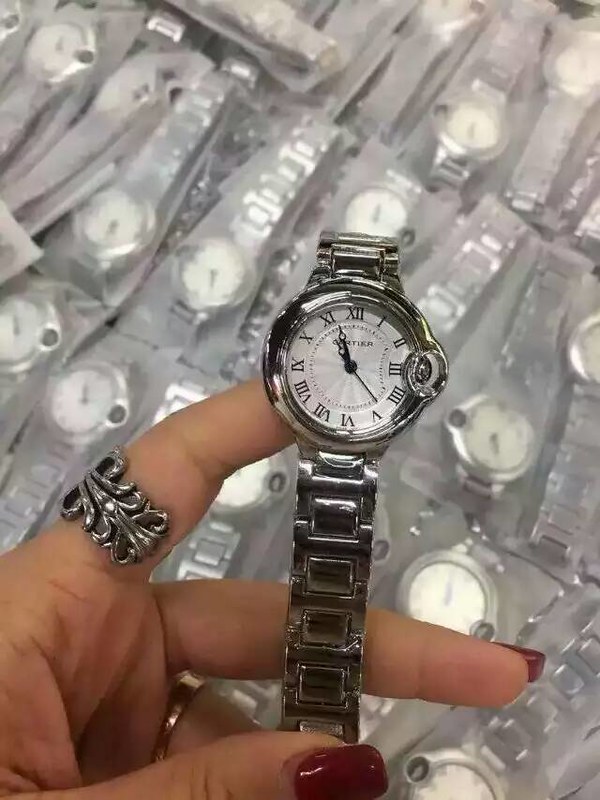This well-lit, indoor color photograph captures the close-up of a lady holding a silver watch at the center of the image. The watch, featuring a stainless steel color and a round body, is being held by the woman's left hand. She grasps the silver band between her thumb and index finger, with her index finger extended behind the watch face. The face of the watch is white with Roman numerals, and it shows a time of approximately 10:55, with the second hand pointing to the 5 o'clock position. Notably, there is a fisheye lens-like bulge where the date is displayed. The woman's red nail polish and a distinctive silver ring on her left index finger are clearly visible. The background consists of neatly arranged rows of similar watches, wrapped in white plastic, giving the impression of a watch shop specializing in mass-produced, potentially knockoff items. The image is in good focus, with no text or print present.